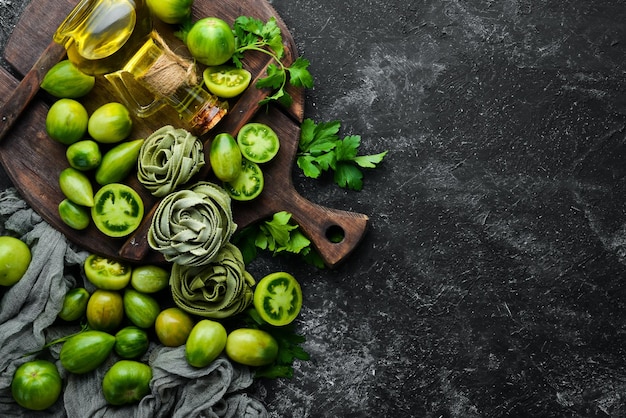The image captures an overhead view of a rustic kitchen scene set against a black and white stone or granite countertop. Dominating the center is a small, wooden cutting board with a handle, displaying several vibrant green tomatillos, a couple of which are sliced open to reveal their interiors. Scattered around the cutting board are more whole tomatillos, a few limes, and sprigs of fresh cilantro. Adding to the arrangement, there's a peculiar glass bottle, possibly containing olive oil, positioned alongside a green, spiral object that might be cloth or noodles. Also present in the scene are three green, flower-patterned towels, creating a soft contrast to the array of produce. The setup is visually complemented by a blue crinkled cloth, contributing to the overall rustic and homey ambiance.